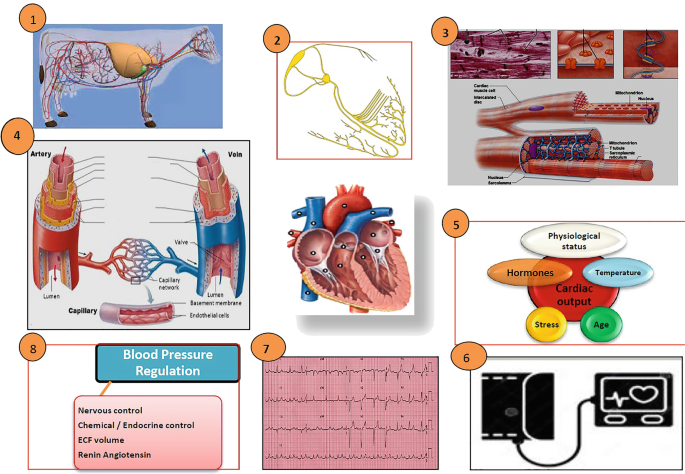The image is a comprehensive, grid-style collage of eight medical diagrams typically found in a doctor’s office or classroom. The upper-left diagram showcases a cross-sectional view of a cow with its circulatory system displayed, including red and blue veins. The diagram next to it features a yellow lattice network, likely depicting the lymphatic system. The third image on the top row is a detailed sketch of blood vessels, with additional microscopic elements that could represent transport proteins. The fourth image in this row elaborates on arterial and venous structures. The centerpiece on the second row provides a cross-sectional view of a human heart, highlighting its chambers and connecting veins and arteries. Adjacent is a bubble diagram with a red circle labeled "cardiac output," surrounded by influences like "age," "stress," "temperature," "physiological status," and "hormones." Below this, the left side of the final row features a diagram titled "blood pressure regulation," detailing mechanisms like nervous and chemical endocrine control, ECF volume, and the renin-angiotensin system. The central image in this row appears to be an EKG graph displaying cardiac rhythms. Lastly, the rightmost diagram depicts a heart monitor setup, including a blood pressure cuff and a screen showing cardiac rhythm.